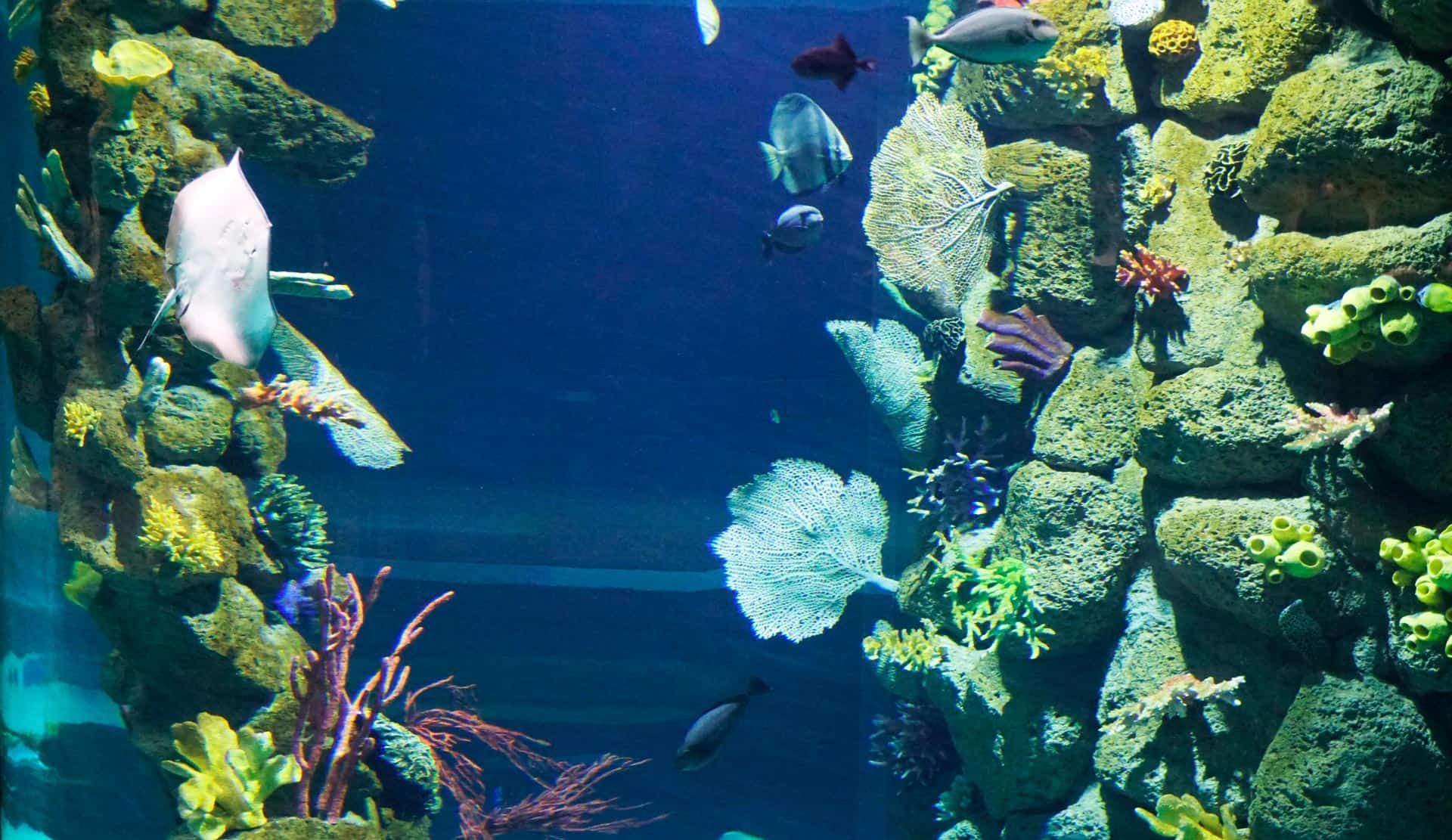This is a highly detailed photograph of an underwater scene taken inside an aquarium. The image captures a vibrant and serene underwater landscape, dominated by coral reefs on both the right and left sides, while the center features the deep blue ocean water. The coral reefs are richly colored with shades of yellow, green, red, purple, and pink, adorned with various rocks and plants, including waving green seagrass. Several fish of different species and colors, ranging from deep black-blue to lighter shades of white, swim around the scene, adding to the dynamic beauty of the photograph. The ocean floor is vaguely visible in the background and lighter portions can be seen in the lower third of the picture. Additional details, like the aquarium glass and structural lines in the background, suggest that the photo was taken indoors rather than in the open ocean. Overall, the image beautifully encapsulates the vibrant and diverse marine life within an aquarium setting.